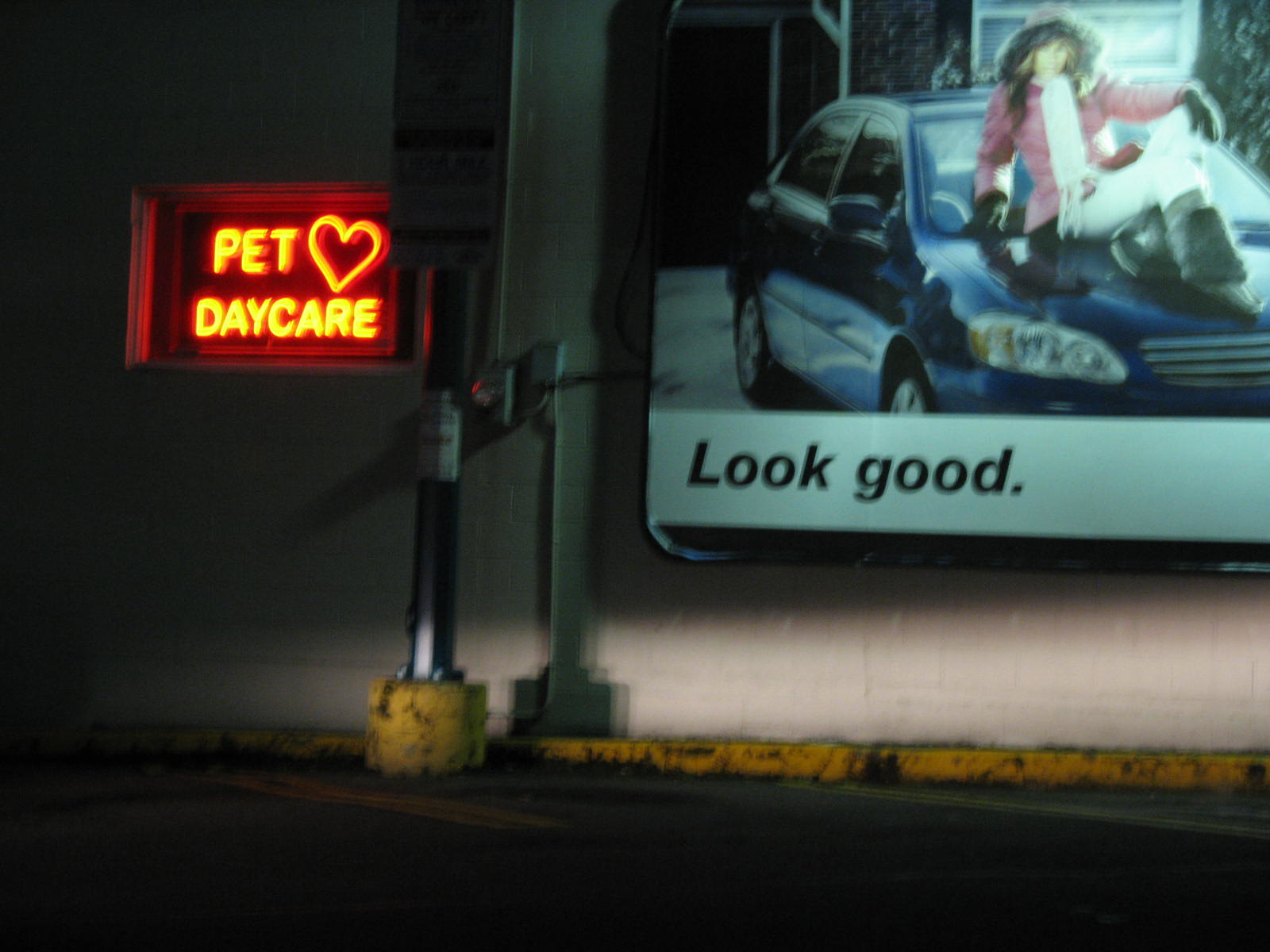This photograph captures a nocturnal scene likely in a street or parking lot area. Dominating the image is a large billboard affixed to a cream-colored cinder block wall, brightly lit against the night. The billboard features an advertisement with the slogan "Look Good Simply" in bold black letters on a white background. The central figure in the advertisement is a woman dressed for winter in a red parka with a fur-lined hood, white pants, winter boots, and snow gloves. She is seated on the bonnet of a blue sedan, which appears to be a regular-looking car.

Adjacent to the billboard on the wall is a smaller neon sign framed in a black background with a silver border. This sign reads "Pet Daycare" in a vibrant red-orange neon font, complete with a heart symbol. Beneath the signage, there is a yellow-painted curb, showing signs of wear, and the blacktop surface of the parking lot.

In the foreground, emerging from a yellow-painted metal base, stands a black metal pole, possibly part of a crosswalk or street fixture. Nearby, a metallic conduit runs along the wall, blending in with its cream color. This detailed night-time scene is visually divided between the striking commercial billboards and the gritty urban textures of the parking area.